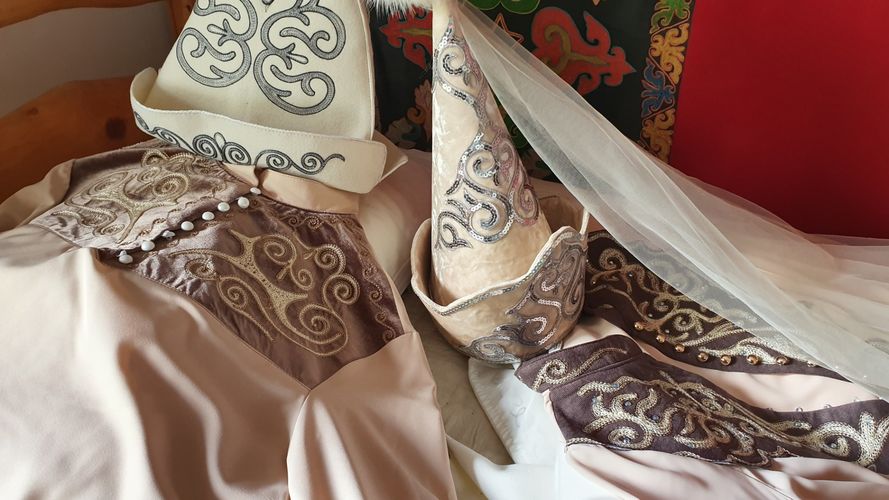The image depicts a close-up of two ornate, decorative shirts laid out on a bed against a red wall backdrop. The shirts are made from luxurious fabric, appearing to be silk with intricate detailing. The primary fabric is a lavender color with delicate dark purple swirls, and the shirts feature small white buttons that run up to the collar. Each shirt is adorned with opulent decorations: white beads along the center and faded red portions with white designs. The elaborate detailing continues with green, yellow, and blue designs on the edges, and red leaf-shaped patterns with yellow lines inside. At the top of each shirt, there is a crown-like, tannish white ornate piece with gray, circular and swerving designs, resembling pointed hats or cones with silver lace and rhinestone swirls extending up from the base. Some sections also have gold balls attached, adding to the richness of the attire.